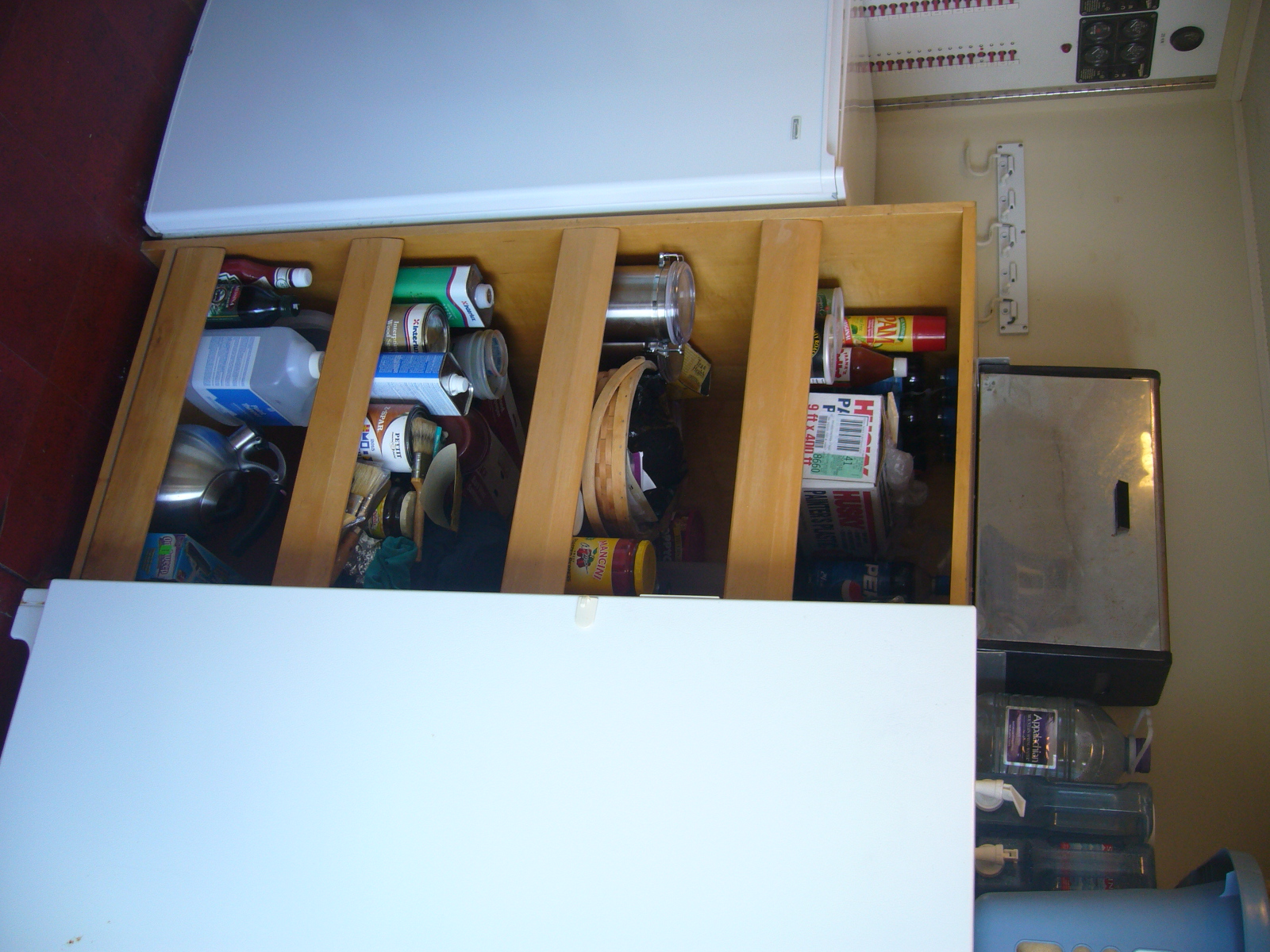This image depicts a close-up view of a cozy kitchen corner, originally taken vertically but meant to be horizontal. The focus is on a wooden countertop surrounded by four sets of open shelving filled with various kitchen utensils and storage items. Among the shelves, you can see kettles, wicker baskets, pans, and containers filled with assorted items. Prominently displayed is a small refrigerator next to light-colored wood shelving. On the countertop, there's a visible toaster, a bread box, a coffee maker, and additional containers. The cream-colored walls behind the setup feature white hooks and possibly a kitchen tool or decoration mounted against them. The flooring appears to be either wooden or designed to mimic a professional kitchen style with a rich red hue. Adding a casual, lived-in touch, a bottle of ketchup is also visible among the array of large-sized kitchen essentials.